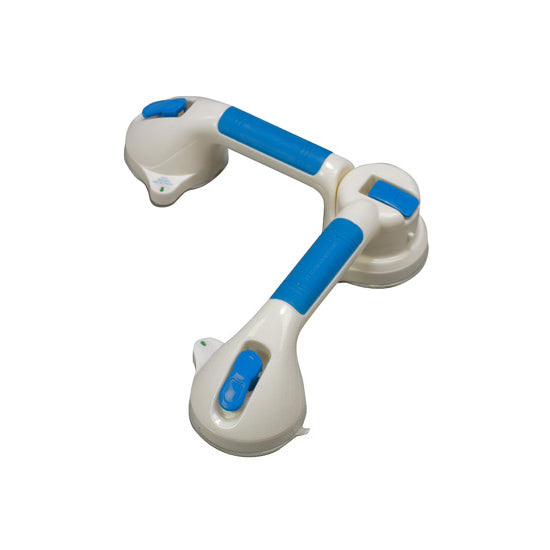The image depicts a white plastic bathroom assistive grab bar designed to aid individuals in getting up from a toilet or bathtub, or maintaining balance. The grab bar features blue grippy surfaces on the handles and blue latches that control the suction mechanism, which help secure the device to a wall. The bar is positioned directly in the center of the image, with parts extending to the bottom left and bottom right. A joint or hinge in the middle suggests it can rotate or change position for adjustable support. The background is entirely white, emphasizing the product and its functional design elements.